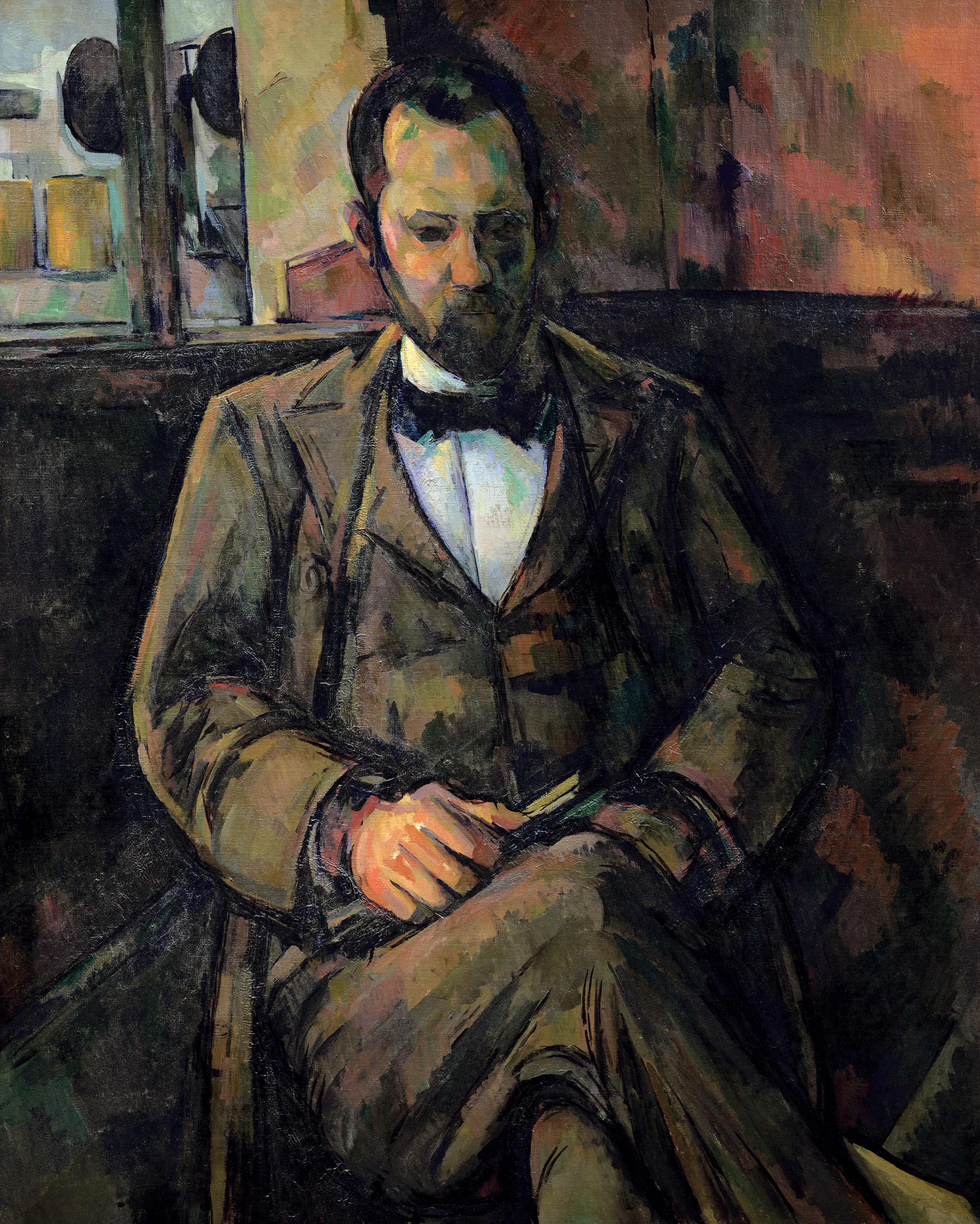This detailed oil painting depicts a solemn man sitting cross-legged on a brown sectional couch, gazing pensively down at a book held in his hands. The man has short, dark hair with a widow's peak indicating slight balding, and sports a full, well-trimmed beard and mustache. He is dressed in a long black trench coat layered over a black blazer, a white dress shirt, and a brown bow tie, matched with dark brown pants. The background features tan walls with dynamic red and black brush strokes. Over his left shoulder, there is a noticeable power pole with round speakers extending from it. Additionally, in the upper left corner of the background, a silver train with small square windows can be seen, adding an intricate detail to the setting. The painting employs muted tones, giving it a contemplative and subdued atmosphere.